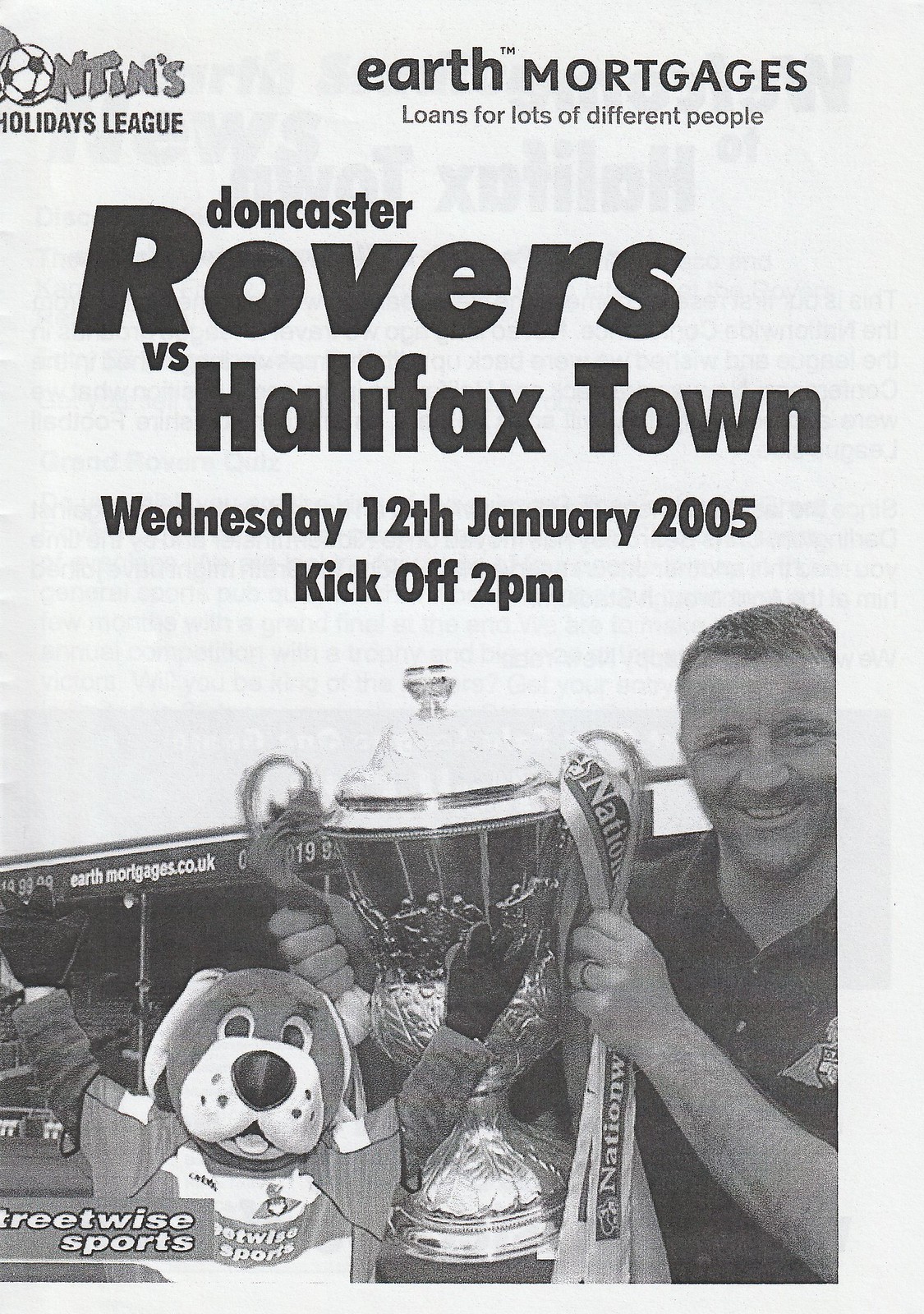The grayscale magazine cover features a prominent advertisement for an upcoming soccer match. At the very top left, partially cut off, is a logo incorporating a soccer ball in place of the "O" followed by “Holidays League.” Adjacent to it on the right, it reads, “Earth Mortgages, loans for lots of different people.” Dominating the central portion of the cover in large, bold black letters is the announcement: "Doncaster Rovers vs Halifax Town, Wednesday 12th January 2005, kickoff 2 p.m." 

Below this central text, positioned towards the right, is a detailed photograph of a man dressed in a collared shirt adorned with a logo, triumphantly holding a large trophy cup intertwined with ribbons. Beside this image is a stuffed plush dog, likely the team's mascot, adding a playful touch to the cover. Also included near the image is the text "Streetwise Sports." The grayscale theme with varying shades of black, white, and gray gives the cover a vintage, classic appearance, reminiscent of a promotional program one might receive at a soccer game.